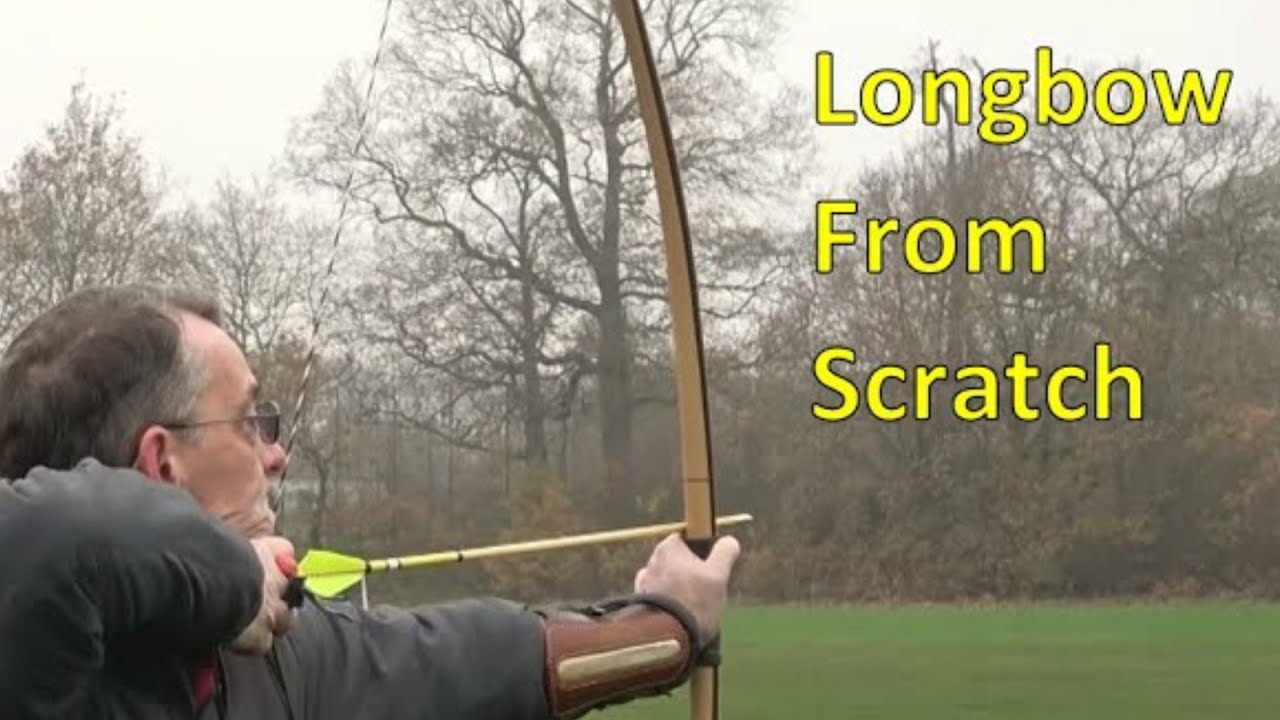In this photograph, we see an older man, likely in his 50s or 60s, pulling back a longbow in a serene, natural setting. Positioned towards the bottom left corner, he is facing the right side of the frame, concentrating intently on the target in the distant, hazy forest backdrop. The man sports a short haircut with graying hair at the temples, a white mustache, and black sunglasses. Dressed in a black sweater, he also wears a leather wrist brace on his left wrist. His right hand pulls the tan-colored arrow back to his ear, showcasing the black-and-white twirling drawstring and bright yellow fletching. The vibrant green, mowed grassy area in the foreground contrasts with the wooded and bushy background under a gray, overcast sky. Large, bright yellow lettering on the right side of the frame reads "Long Bow from Scratch," emphasizing the simplicity and craftsmanship of the bow.